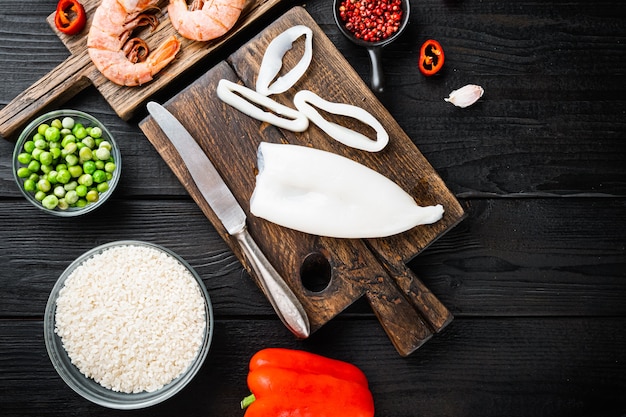The image captures a meticulously arranged scene set up for cooking on a black rustic table, its textured grain visible through the dark paint. Dominating the center is a substantial dark brown wooden cutting board, adorned with cleaned squid, including three neatly sliced rings and a shiny silver knife placed beside them. Positioned diagonally above it is a smaller cutting board bearing at least two large prawns. A variety of ingredients and containers are strategically placed around these boards: to the left, a plastic container holding what looks like green snap peas, and another with white granules resembling finely chopped rice. Below the main cutting board lies a vibrant red bell pepper, while on the upper right corner, there’s a small ramekin filled with pomegranate seeds, flanked by a slice of chili pepper and a garlic clove. Additionally, a black pot sits near the top middle, filled with something red, contributing to the scene's rich array of colors and textures.